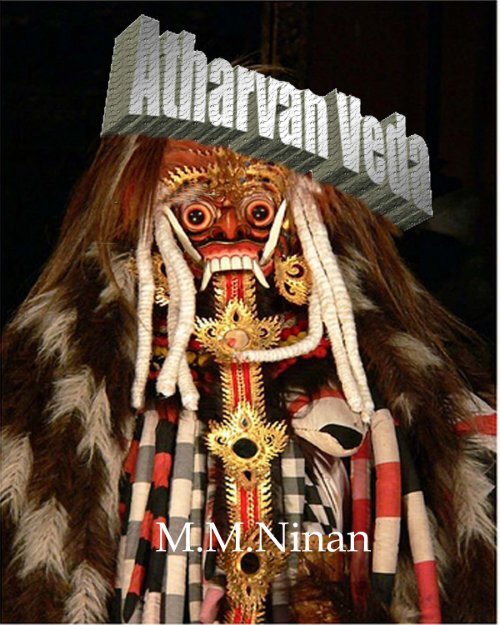The image features a mysterious and eerie creature against a black background. At the top of the image, in bold gray 3D letters, it reads "Atharvan Veda". Below, at the bottom, it says "M.M. Ninan" in white text, presumably indicating the author or creator.

The central figure is an unsettling and complex character that appears to be a ceremonial or tribal entity. The creature's face is adorned with circular red eyes with black centers, and it has a golden pine needle-like arrangement forming its eyebrows. The eyes are described as pure black, giving it a haunting expression.

Its mouth is filled with an array of teeth, including two prominent fangs at the top and bottom. The teeth are both normal flat white teeth and elongated fangs, creating a menacing appearance. The creature's tongue is a striking gold color, with red in the middle and spiky golden projections along its sides, decorated with large gold pendants.

The character's head is topped with long, brown, dreadlock-like hair, interwoven with thick, white ropes and adorned with white and brown feathers on either side, draping down its shoulders. Additionally, it has various striped ropes in white, gray, black, and red colors adding to its intricate appearance.

Altogether, the creature appears as if made from real objects, with meticulous details that create a surreal and terrifying visage.